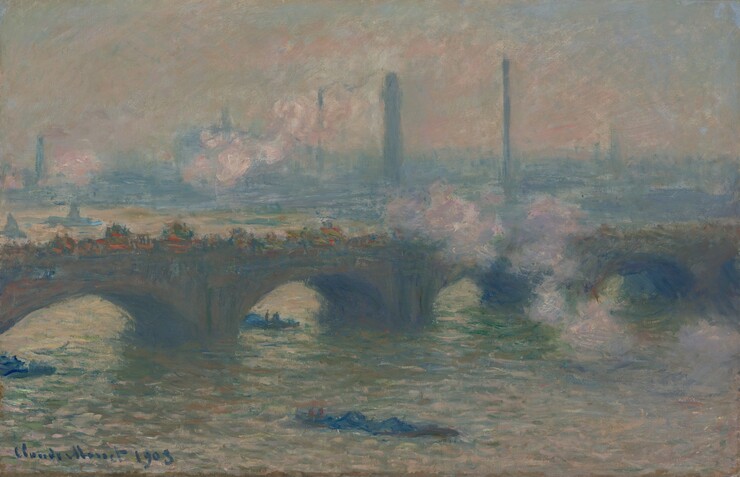The image we're examining is a painting from a historical period, likely depicting an industrial city. The main feature of the artwork is a stone bridge spanning across a river. Below, elongated boats are being rowed through the water. In the background, the cityscape is dominated by smoke stacks emitting large clouds of noxious smoke, enveloping the area in a thick smog, reminiscent of London during the Industrial Revolution when coal was a primary energy source. The sky is filled with dark, oppressive smoke, indicating severe air pollution. The painting employs dark colors and lacks intricate detail, focusing more on the broad, grim atmosphere of industrialization rather than specific elements.